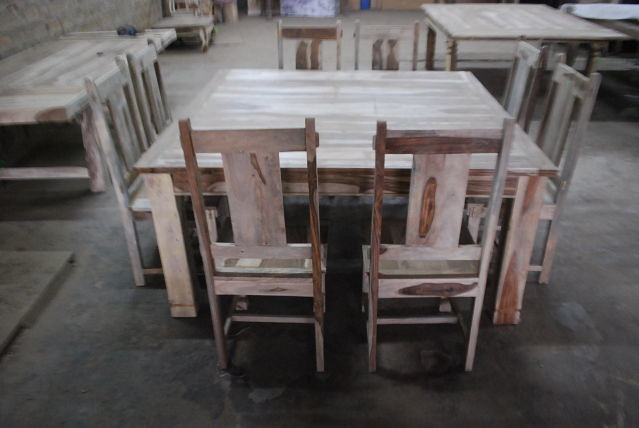This photograph depicts a rustic and vintage-style dining room, featuring an ensemble of wooden tables and chairs with a weathered, antique appearance. The focal point is a large square table positioned centrally, crafted entirely from what appears to be birch wood with a muted grayish-brown hue. It is surrounded on all four sides by eight high-back wooden chairs, two on each side, matching the table in material and aged finish. In the background, the room holds additional wooden tables—three in total—one against a stone wall to the left and another in the far upper right, both without accompanying chairs. The entire setting rests on what seems to be a cement floor, enhancing the room's overall rustic and historical ambiance.